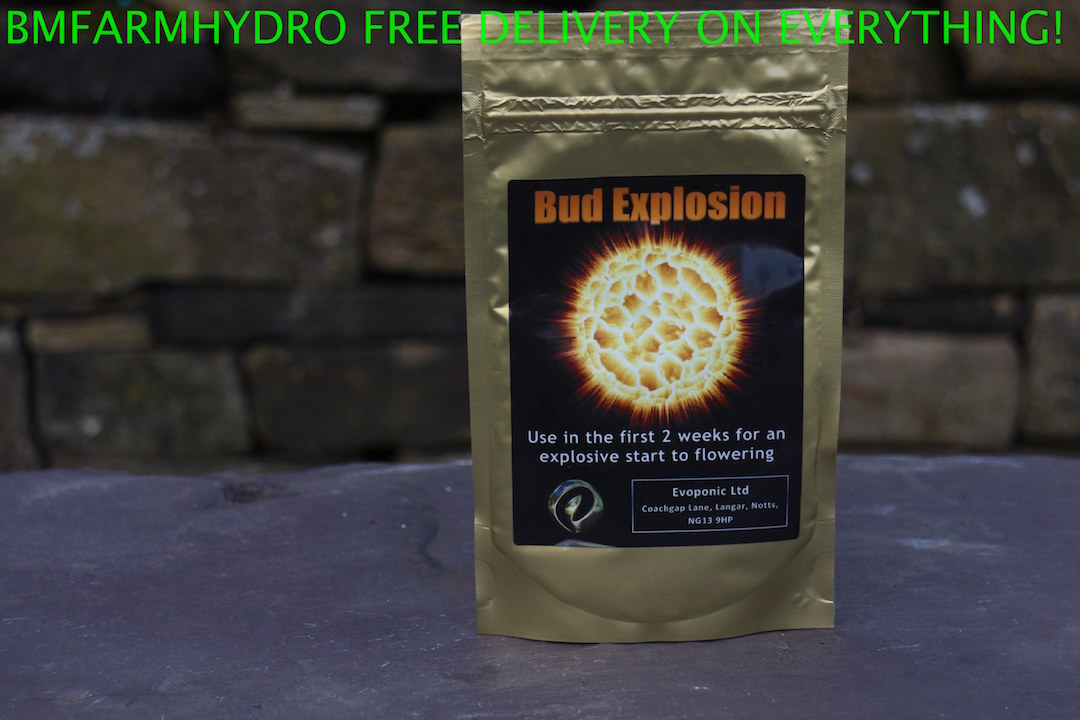The image displays a promotional depiction of a gold-foiled, resealable pouch labeled "Bud Explosion." The pouch sits on a gray stone surface with the backdrop of a greenish-brown brick wall composed of uneven-sized stones. The black label on the pouch features the product name "Bud Explosion" in bold orange letters and a graphic of a marijuana bud emitting radiant, sunburst-like rays. Beneath this, in white text, it instructs: "Use in the first two weeks for an explosive start to flowering." Further below, within a white-bordered rectangle with a black background, the text reads "Evoponic Ltd, Coach Gap Lane, Langer Knots, NG13 9NP." Dominating the top of the image in vibrant green, all-capital letters, it proclaims: "BM Farm Hydro, FREE DELIVERY ON EVERYTHING!"